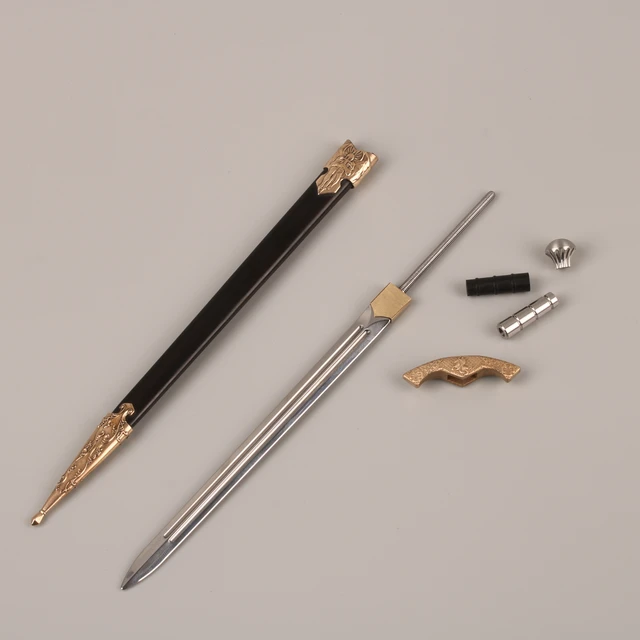The image shows a meticulously arranged set of disassembled components of a pen laid out against a gray background. On the left side, there is a black body part with a gold band at the top and a gold pointed tip at the bottom, resembling a pen's outer casing. Beside it, to the right, lies the internal assembly which includes a cylindrical silver ink refill with a pointed end, a small silver screw, a gold ring, and another black round piece. Further right, there's a metal cap. Each part is clearly visible and distinct, highlighting the intricate design and assembly required for a functional pen.